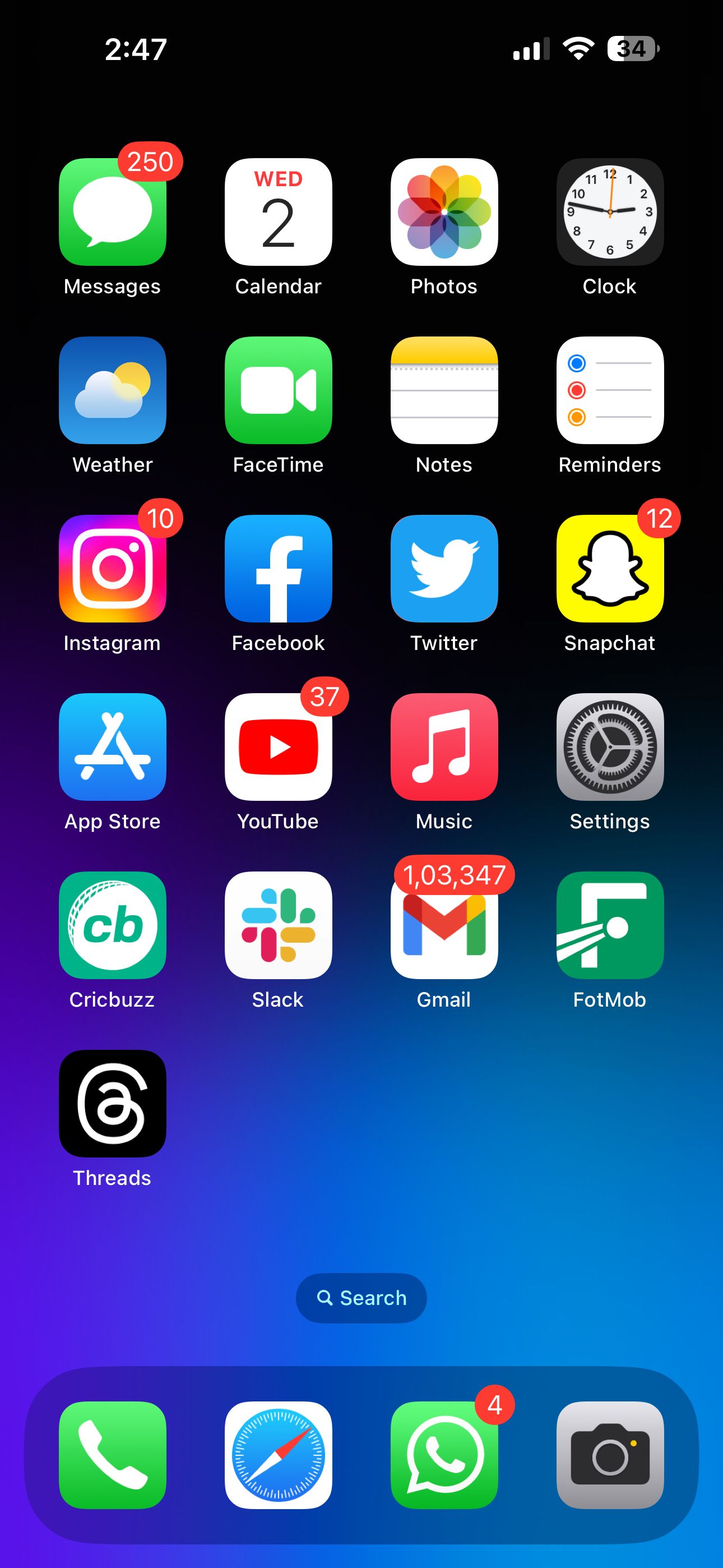A screenshot of an iPhone screen displays various details and apps organized in a grid. In the upper left corner, the time is shown as 2:47. The upper right corner indicates a battery level of 34%, with the Wi-Fi showing full signal strength and three out of four bars for cellular signal.

**First Row of Apps:**
1. Messages - 250 unread messages.
2. Calendar - shows "2" for Wednesday.
3. Photos.
4. Clock - displays 2:47.

**Second Row of Apps:**
1. Weather.
2. FaceTime.
3. Notes.
4. Reminders.

**Third Row of Apps:**
1. Instagram - 10 unread notifications.
2. Facebook.
3. Twitter.
4. Snapchat - 12 unread notifications.

**Fourth Row of Apps:**
1. App Store.
2. YouTube - 37 unread notifications.
3. Music.
4. Settings.

**Fifth Row of Apps:**
1. CrickBuzz.
2. Slack.
3. Gmail - 103,347 unread emails.
4. BotMob.

**Sixth Row:**
- Threads.

At the bottom center is the Search bar, and the dock at the bottom includes:
1. Phone.
2. Safari.
3. WhatsApp - 4 unread notifications.
4. Camera. 

This detailed organization offers a comprehensive look at the user's iPhone home screen and the status of various notifications and messages.